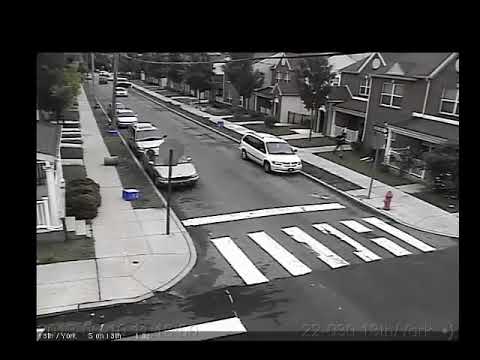This low-resolution, black-and-white photograph, likely taken from a street lamp or security camera, captures a typical American suburban neighborhood. The image shows a road intersecting with another road and a row of two-story houses, each with gray siding and white windows, stretching away into the background along the right side. The houses, positioned closer to the viewer on the right and becoming more distant towards the top left, feature covered porches with white railings and well-manicured lawns. In the foreground, a white sidewalk runs parallel to the road, alongside a couple of trees in the front yards. Prominently, a red fire hydrant stands at the bottom right corner. A black sedan, topped with an open sunroof, is captured driving over a crosswalk on the left side of the photo, while a white van is parked in front of the second house from the right. The overall setting conveys the calm and ordered vibe of suburban life at an intersection.